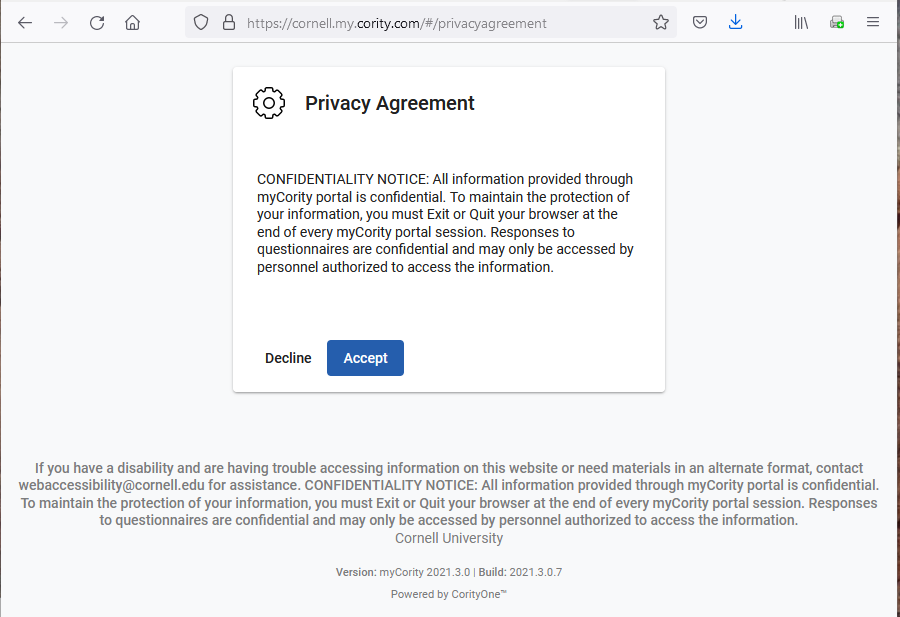**Detailed Description of the Screenshot:**

The screenshot in question is captured from a website interface. At the very top, there's a gray banner adorned with several navigation icons. These include a black left-pointing arrow on the far left, followed by a gray right-pointing arrow right beside it. Next, there's a black refresh icon and a black home icon.

Below the banner, there's a text input space which is currently grayed out and features a URL placeholder for website navigation. To its right is a series of utility icons. First, a blue download button with a downward-pointing arrow, ostensibly paired with what resembles a staple icon underneath. Next, there's a gray icon depicting three stacked lines that look like books, likely indicating a bookmark feature. Following this is a green printer icon, and then a grey icon showing three horizontal lines, which is typically the symbol for a menu or settings.

Dominating the central section of the gray background is a prominent white box. In the upper left corner of this box is a black outlined gear icon, signifying settings or configuration. Adjacent to the gear icon, the text "Privacy Agreement" is prominently displayed. Below it, another heading reads "Confidentiality Notice". The accompanying text states:

"All information provided through my Cornell profile is confidential. To maintain the privacy of your information, you must exit or quit your browser at the end of every myCornell portal session. Responses to questionnaires are confidential and may only be accessed by personnel authorized to access the information."

At the bottom left of this white box are two buttons: a black "Decline" button and, to its right, a blue "Accept" button with white text. Beneath this, in gray text, there's a footer message that reads:

"If you have a disability or are having trouble accessing information on this website or need materials in an alternate form, contact webaccessories@cornell.edu for assistance."

The message reiterates the importance of maintaining confidentiality by exiting or quitting your browser after using the portal to protect your information.